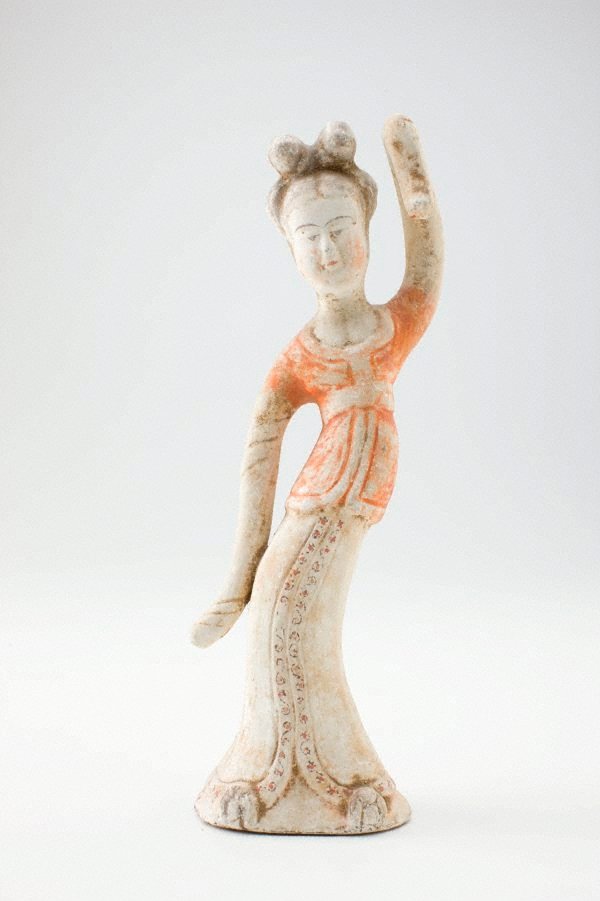This is a horizontal, rectangular color photograph featuring an ancient, oriental-style ceramic figurine. The background transitions from a whitish hue at the bottom to a darker gray at the top. The statue depicts a dancing woman, made of light-colored pottery or stone speckled with brown. She stands on a rounded base, with her left arm raised gracefully above her head, possibly broken at the top, and her right arm resting lower. She is dressed in a long, orange or pink jacket with a white skirt adorned with decorations on the front, suggestive of figures or characters. Her bare legs are visible at the bottom. The figurine showcases detailed facial features including dark eyebrows and a pink mouth, enhanced by her dark brown hair styled with two prominent bones or protuberances on top. Her hair appears to be wrapped in a scarf, completing the intricate details of this evocative piece.